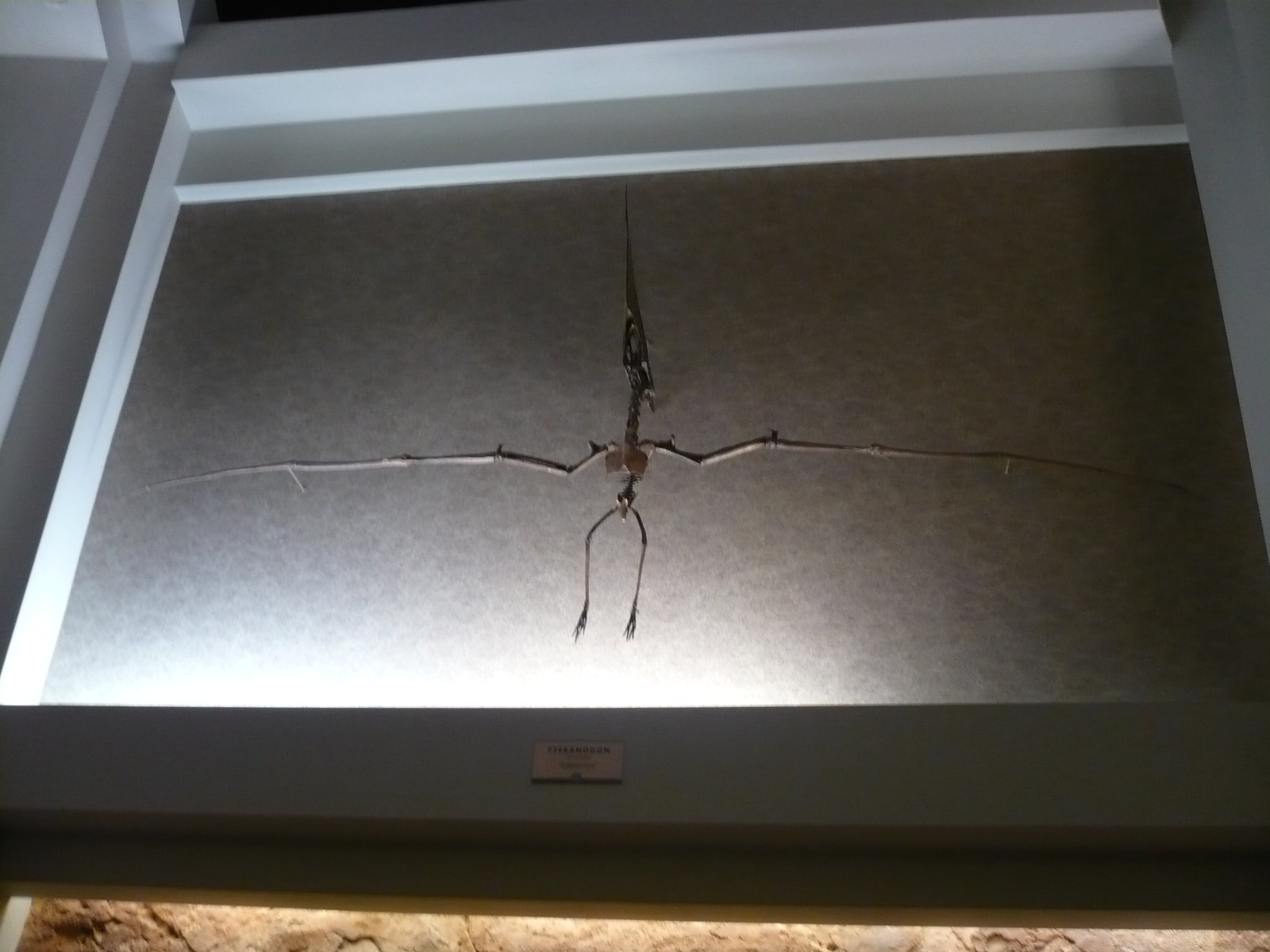The image depicts a museum display of a pterodactyl skeleton, encased within a white-framed glass case, set against a pebble-textured and whitish background, possibly illuminated from the bottom. The skeleton features an elongated skull with a long, pointed bony crest, nearly matching the length of its body. Its rib cage, spine, pelvis, and long, slender legs are clearly visible. The pterodactyl’s most distinctive feature is its expansive wingspan, characterized by extremely long arms with joints at the shoulders and elbows, and elongated hand or finger joints extending from the wrists. The skeleton's color is gray, contrasting with the white trim and the wooden bordering of the display case. Centrally positioned within the frame, the exhibit is accompanied by a small, hard-to-read plaque at the bottom, and it appears against a gray stone wall.